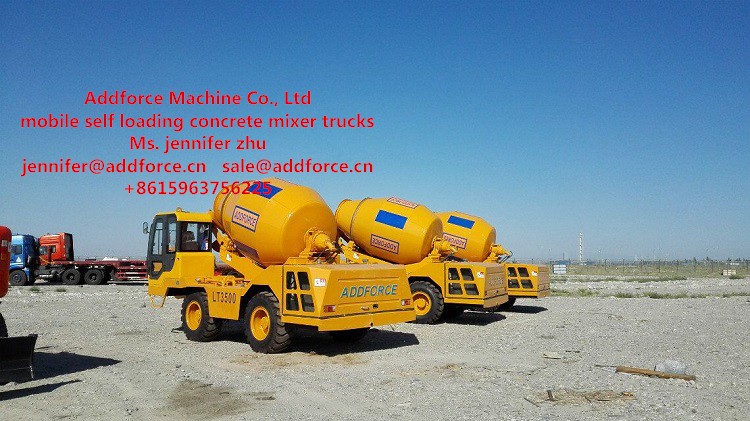The image captures a sprawling dirt lot set against a clear blue sky, filled with heavy construction equipment. To the left, there are two semi-trucks with flatbeds; one features a red cab while the other has a blue cab. Centrally positioned are three prominent yellow cement trucks, each adorned with blue and pink stripes and labeled with "ADFORCE" in black text. The nearest cement mixer displays "LT3500" on its side. Additionally, red text at the top of the photograph reads, "ADFORCE Machine Company, LTD, Mobile Self-Loading Concrete Mixer Trucks, Ms. Jennifer Zhu, Jennifer at adforce.cn, sale at adforce.cn, plus 861-596-375-6225." The vast lot is primarily gravel with some scattered poles and patches of grass, giving a stark industrial feel with no buildings in sight.